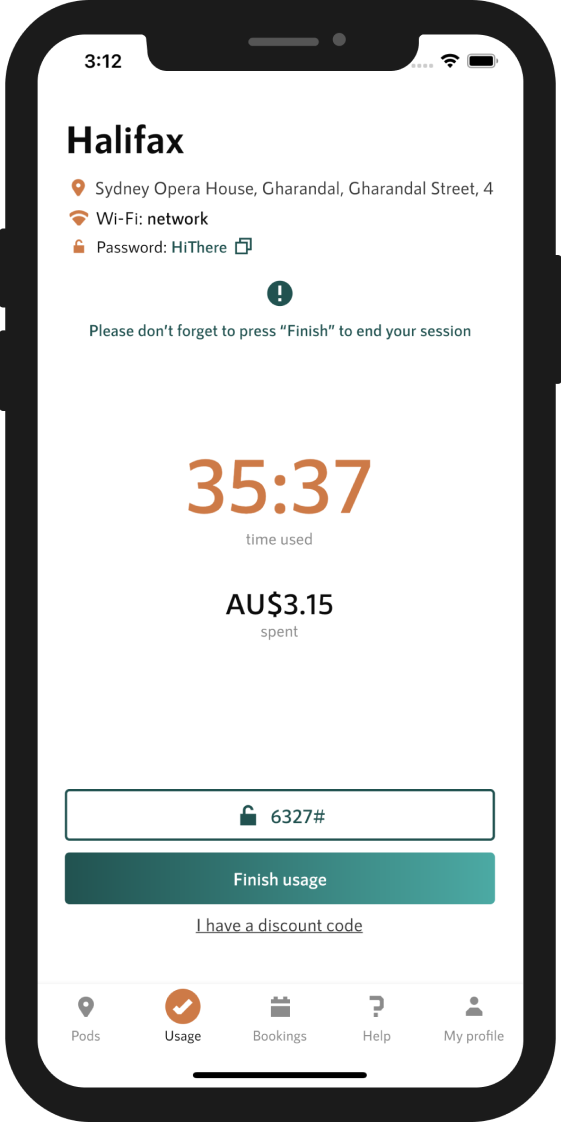The image depicts a smartphone screen with the following details:

- **Top Section:**
  - **Top Left Corner:** Displays the time "3:12."
  - **Top Right Corner:** Shows a full WiFi signal and a fully charged battery icon.

- **Header:**
  - Beneath the status bar, on the left side, are bold black letters spelling out "Halifax."

- **Location Information:**
  - Below "Halifax," a location pin icon is present, followed by the text "Sydney Opera House, Garendall Street 4."

- **WiFi Network Details:**
  - Under the location information, there's a WiFi icon accompanied by the text "Wi-Fi network."

- **Password Information:**
  - Following the WiFi network details is a lock icon accompanied by the text "Password: hi there" and a "Copy hyperlink" option next to it.

- **Session Reminder:**
  - Next, there's a black circle with a white exclamation mark. Below this circle, the text reads "Please don't forget to press finish to end your session."

- **Usage Information:**
  - Below the session reminder, brown numbers "35:37" are displayed, which likely indicates the time elapsed.
  - Following the duration, small gray letters state "Time used."
  - At the bottom, in capital black letters, the cost is displayed as "AU$ 3.15."